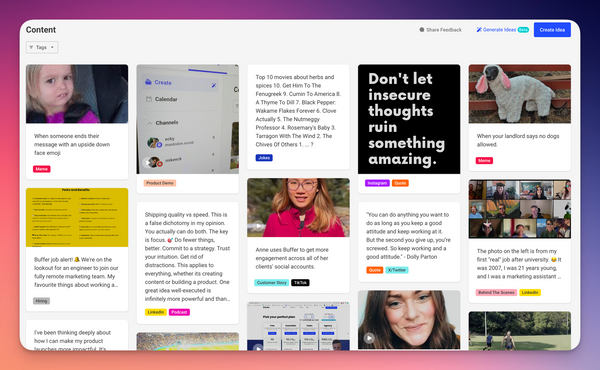The webpage showcases a grid of various thumbnails, each potentially representing articles, memes, or other clickable content. The layout is framed with a gradient border transitioning from peach at the bottom left to purple at the top right. The word "Content" is prominently displayed in the top left corner, while a blue clickable link, housed in a blue box, is positioned at the top right, though the text within the link is unclear.

The main area features approximately ten items, though some are partially obscured. One notable thumbnail, located second from the top right, reads: "Don't let insecure thoughts ruin something amazing." This item includes two descriptors at the bottom, likely indicating the categories it belongs to.

A standout meme in the top right corner depicts an animal dressed as a sheep with the caption: "When your landlord says no dogs allowed," suggesting it's a dog disguised in a sheep costume. Overall, the page appears to be a collection of humorous and engaging content.